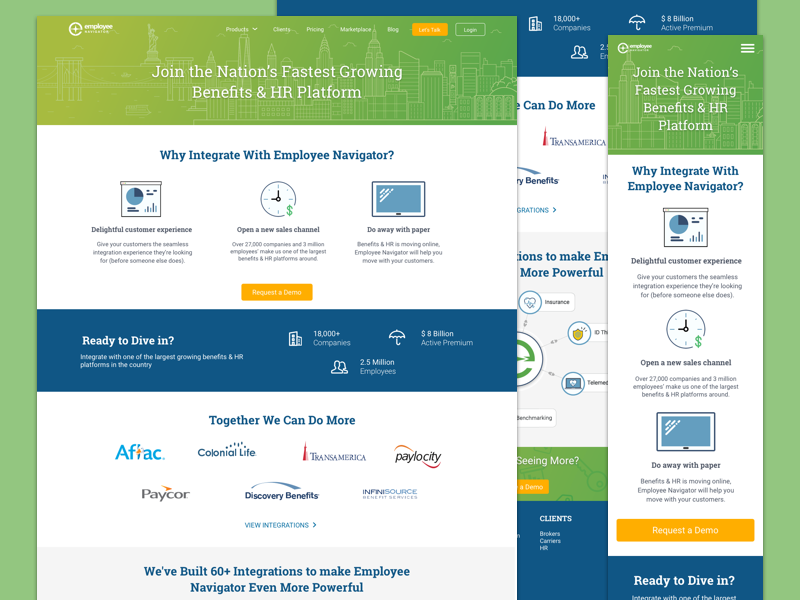A detailed and precise caption for the image could be:

"The web page features a vibrant design dominated by green, yellow, blue, white, and some red accents. At the top, there is a circular logo with a cross, labeled 'Employee'. The prominent header reads, 'Join the Nation's Fastest Growing Benefits and HR Platform'. A green banner showcases a New York City skyline, complete with icons like the Statue of Liberty and the Empire State Building. An orange button labeled 'Let's Talk' stands out against this backdrop. Below, a white banner with blue text offers a 'Login' option and asks 'Why Integrate with Employee Navigator?' Adjacent to it, another orange button invites visitors to 'Request a Demo'. Further down, a blue banner asks 'Ready to Dive In?' and features an umbrella graphic alongside impressive statistics: '8 Billion Active Premium' and '2.5 Million Employees'. A motivational message, 'Together We Can Do More', appears in blue text. The page also displays recognizable logos such as AFLEC, Colonial Life, Transamerica, Paylocity, Paycor, Discovery Benefits, and Infinisource. To reinforce its value, a statement in blue writing announces, 'We Built 60+ Integrations to Make Employee Navigator Even More Powerful'."